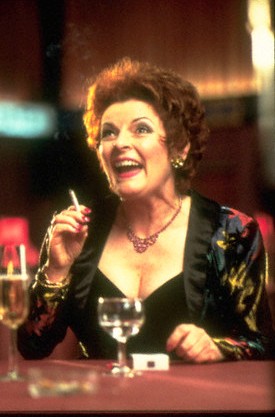The image depicts a woman seated behind a red table, captured from just below her chest upwards in a horizontal rectangle. She is slightly turned to her left, her mouth open in laughter, revealing her top teeth. With medium-length reddish-brown hair, she exudes a lively and engaging presence.

The woman is adorned in a shiny black outfit with a multicolored, possibly gold and red, robe draped over it. Her undershirt features a low-cut V-neck. She accessorizes with a necklace and earrings. In front of her, her left hand rests on the table, while her right hand is bent at the elbow, holding a cigarette up towards her face.

On the table, positioned in the foreground, there's a glass to the left and a goblet directly in front of her. Nearby, to the right of the goblet, appears to be a pack of cigarettes. The background is blurred, hinting at a couple of walls with varied coloration, predominantly shades of red and beige.